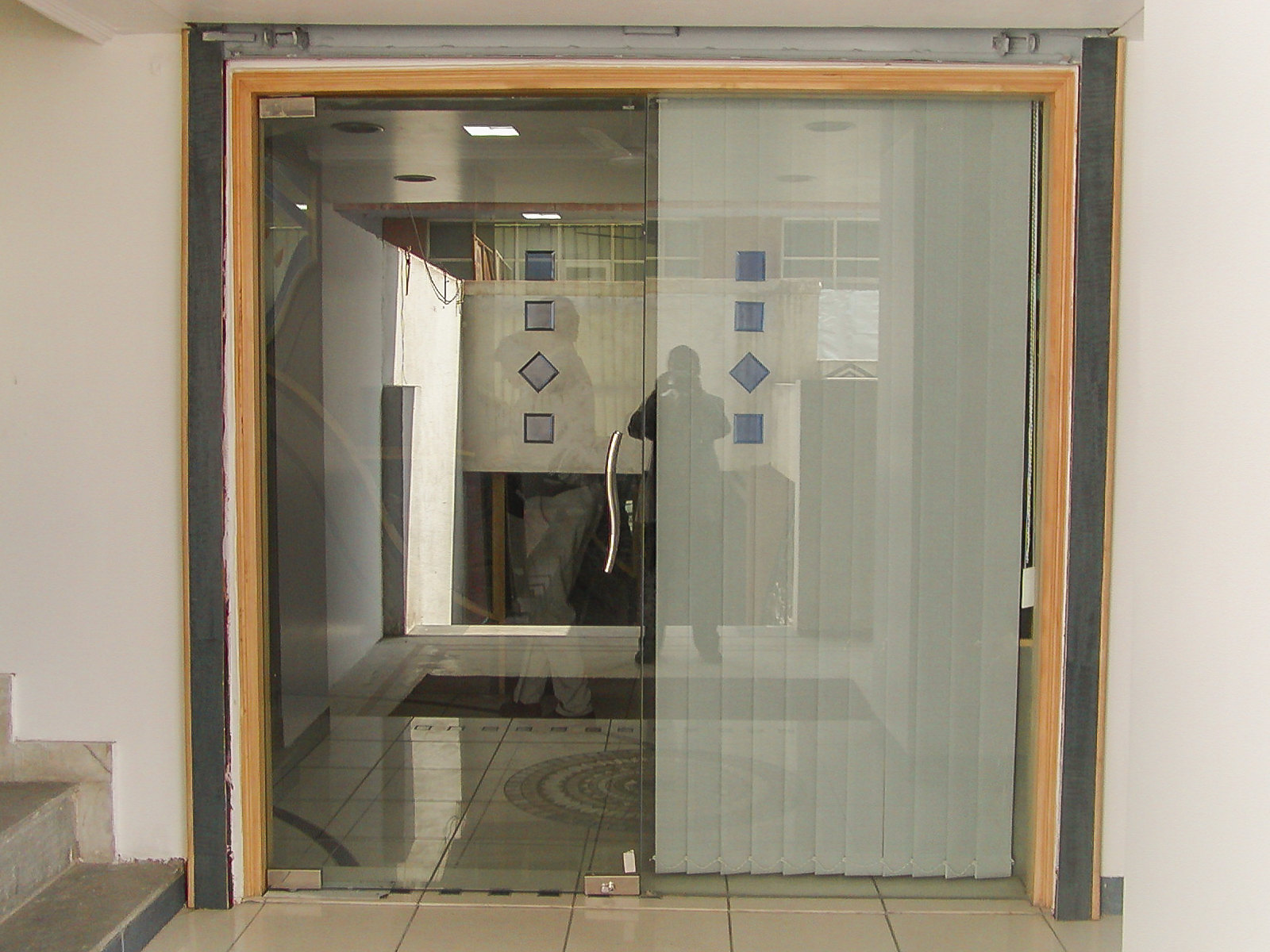The photograph, rectangular in shape, captures an indoor scene focusing on a set of sliding glass doors framed in honey-colored wood. The right-hand door panel is covered by closed white vertical blinds, while the left-hand panel is clear, revealing some of the room beyond, along with reflective views of the interior space. The reflection on the glass shows a patterned tile floor with circular designs and glimpses of the photographer, who appears to be wearing a dark suit. Additional details include square and diamond-shaped patterns in the wall tiles behind the photographer. Adjacent to the left of the glass doors, a set of tiled concrete steps ascend, and the surrounding walls are painted an off-white color. The doors also feature visible metal fittings and a sliding mechanism at the top.